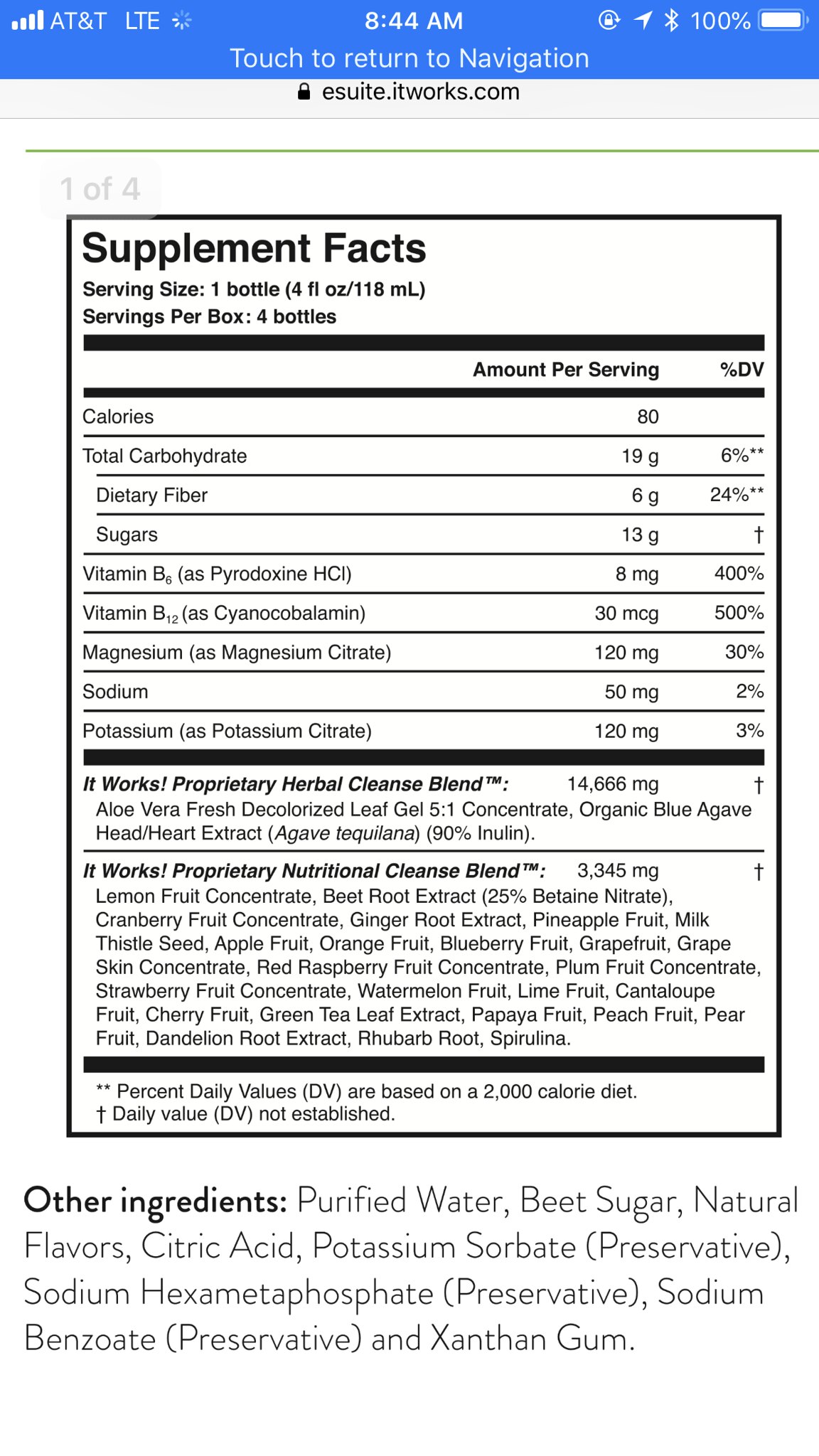This image is a screenshot captured from a mobile device that displays the nutrition label of an unidentified product. The screenshot, taken at 8:44 a.m., reveals that the user accessed the information through the website esuite.itworks.com. The label itself pertains to a dietary supplement, encapsulated in a single bottle, with detailed nutritional information and an ingredient list.

The nutrition facts section comprises standard nutritional values such as calories and carbohydrates. The ingredient list is notably thorough, including water, beet sugar, natural flavors, citric acid, a variety of preservatives, and xanthan gum. This comprehensive label gives a clear insight into the nutritional composition and ingredients of the supplement, despite the product itself remaining unidentified.